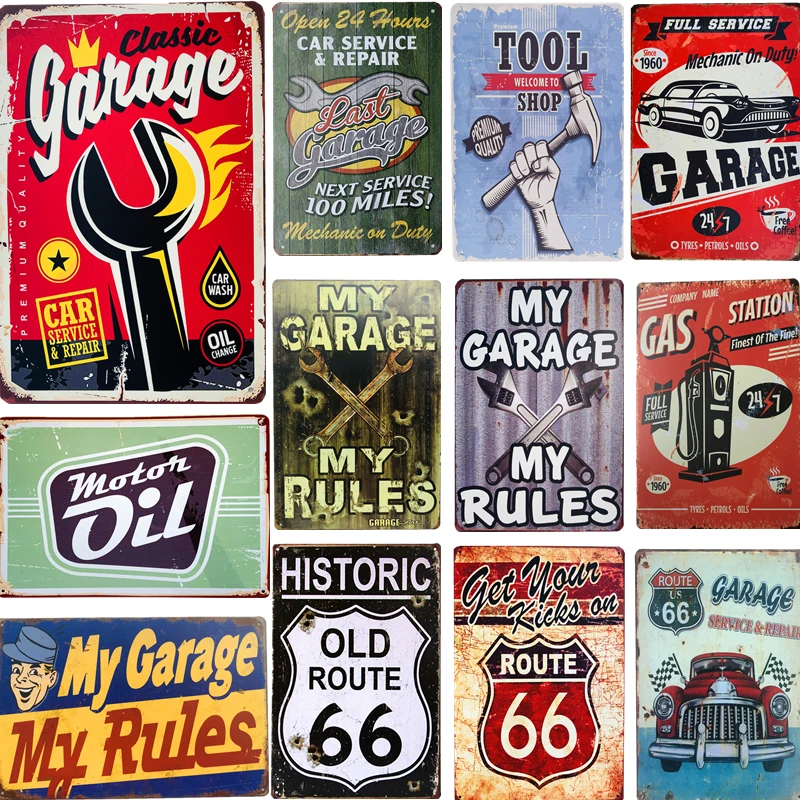The image showcases a vintage-themed wall adorned with 12 old-fashioned signs, primarily related to auto repairs and garages, exuding a nostalgic charm. Prominent signs include one with a hand holding a hammer, labeled "Premium Quality," and another in the upper left corner saying "Classic Garage" with a red background and a crown. There are multiple Route 66 references, such as "Historic Old Route 66," "Get Your Kicks on Route 66," and "Garage Route 66." One notable sign features a giant wrench with flames, reading "Car Wash Oil Change," while another green and oblong-shaped sign states "Motor Oil." Additionally, there are multiple occurrences of "My Garage, My Rules," some with crossed wrenches and varying conditions of rustiness. Other details include a sign indicating "Full Service Gas Station," "Mechanic on Duty Garage 24-7," and "Next Service 100 Miles." The signs, with their varied hues of red, green, and blue, along with their vintage design elements, create a cohesive display that vividly recalls the bygone era of classic car service stations.